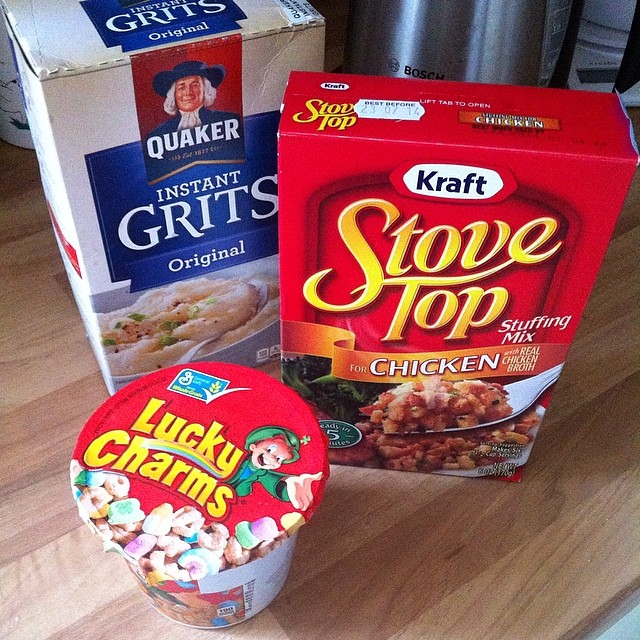The image depicts a wooden table with a light to medium brown hue, on which three food item packages are arranged. At the forefront is an individual-use container of Lucky Charms cereal. The package, designed as its own bowl, prominently features the iconic leprechaun mascot in a green hat and jacket, along with colorful marshmallows, and "Lucky Charms" written in bright yellow lettering on a red background. The second item is a box of Stove Top Chicken flavored stuffing mix by Kraft. This red box showcases "Stove Top" in large yellow letters, "stuffing mix" in white, and an image of brown stuffing with a silver fork and green broccoli. Behind these two is a large, white rectangular box of Quaker Instant Grits Original. This package includes an image of the Quaker man with a blue hat and jacket and a white ruffled shirt. "Quaker Instant Grits Original" is clearly stated across a blue label with "Grits" in large white letters, accompanied by a photograph of creamy grits garnished with green onions in a white bowl with a silver spoon.